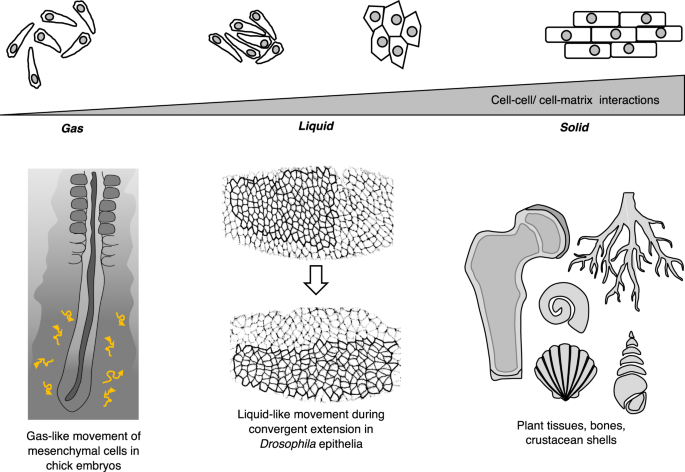This detailed black-and-white illustration, reminiscent of a textbook diagram, visually explains the transition and movement of cells in different states of matter. At the top, it showcases the arrangement of particles in gas, liquid, and solid states, with accompanying labels: "Gas," "Liquid," and "Solid." Above the depiction of solid-state particles, the annotation reads "cell-cell / cell-matrix interactions," elucidating how individual cells interact within the matrix. Below this sequence, the illustration breaks down into three specific examples of cellular movements. To the left, a caption states "gas-like movement of mesenchymal cells in chick embryos," accompanied by relevant imagery. Centrally, the diagram highlights "liquid-like movement during convergent extension in Drosophila epithelia," and on the far right, it depicts "plant tissues, bones, crustacean shells," with visual representations of shells and bones, drawing connections between different biological materials and their structural dynamics.